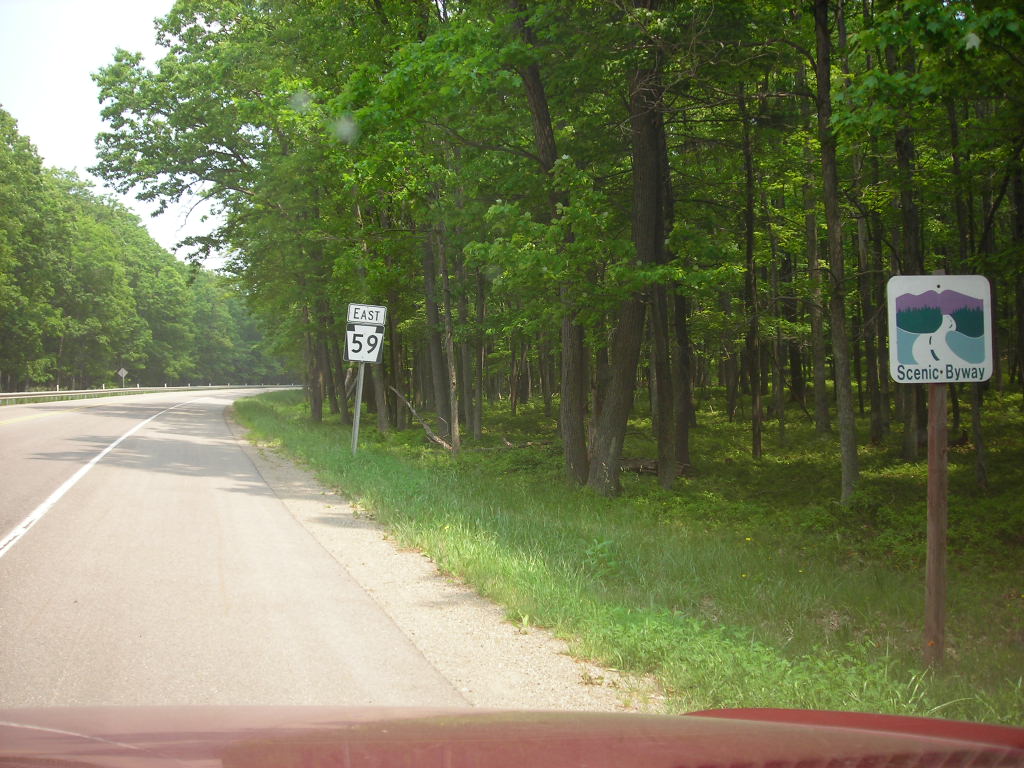This vibrant photo, taken from the dashboard of a red vehicle, captures a sun-drenched summer day on a picturesque, curved road. The vehicle's red hood forms a striking contrast against the lush surroundings. A solid white centerline guides the way, while a sturdy guardrail runs along the left side of the road, protecting against the forested drop-off. The road is flanked by verdant grass that transitions seamlessly into a dense array of tall, leafy trees, their shadows playfully dancing on the pavement. Above these trees, a sliver of blue sky is visible, adding depth to the scene. Two distinct signs stand out: one promoting the Scenic Byway with an illustration of purple mountains and a winding road, and the other indicating the route as East 59. The image perfectly captures the beauty and serenity of a leisurely summer drive through nature.